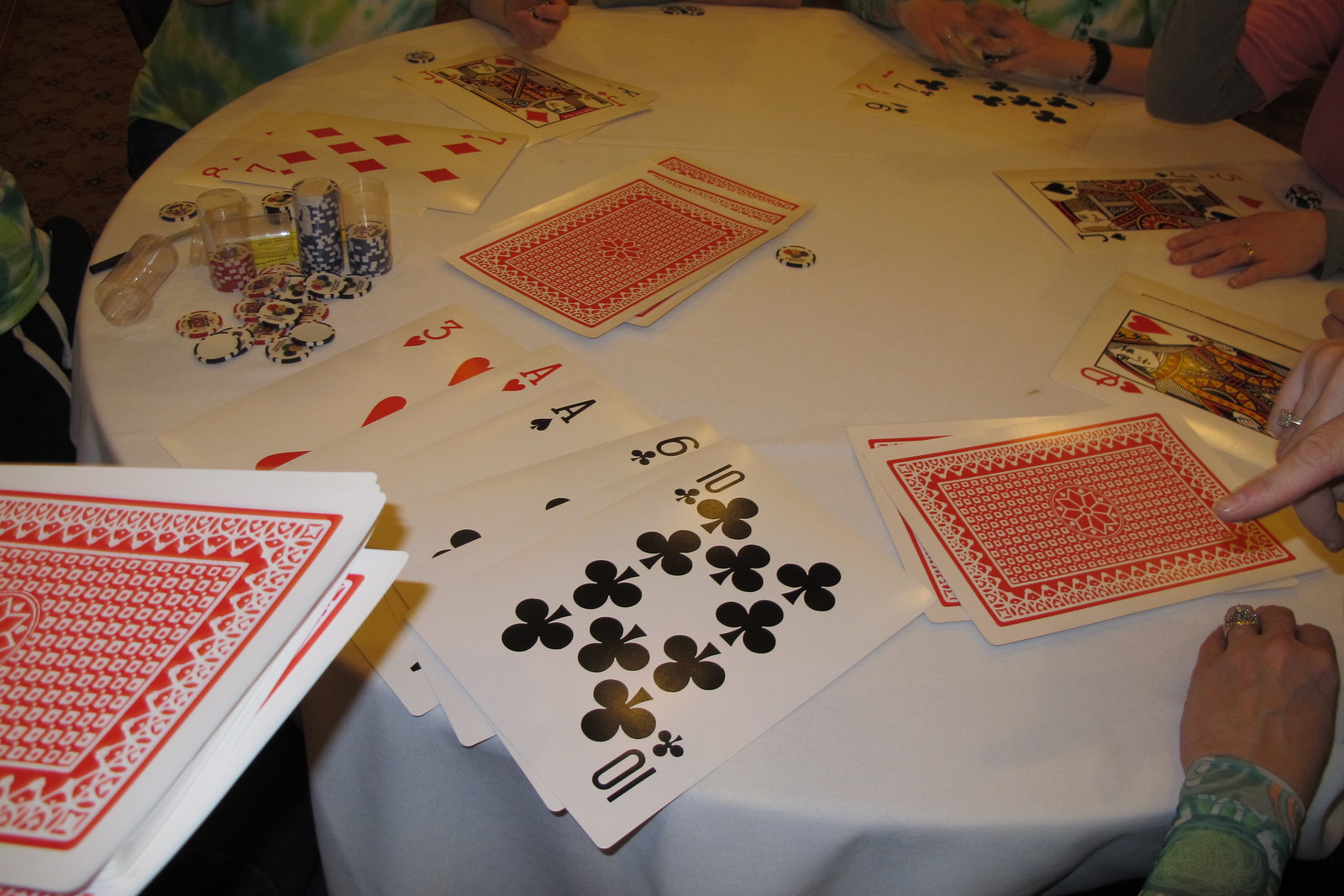In the image, we observe a round table draped with a pristine white tablecloth, around which several individuals are seated. Each person has oversized playing cards laid out in front of them. The backs of the cards are decorated with a red and white design, while the faces exhibit the traditional playing card symbols in red and black. Scattered on the table are betting chips, some still encased in plastic containers. The hands of the participants, likely belonging to older Caucasian individuals based on visual clues, display wedding rings and wristwatches.

The arrangement of the cards suggests they are in the midst of a game or have just completed a round; some cards lie face up, while others remain face down. Close to the camera, the visible cards include a three, two aces, a six, a ten, and a partially concealed card under the ten. As we scan around the table, we can identify more cards: a seven, eight, joker, king, another seven, two, nine, joker, three, and queen. One player maintains their cards face down, adding a dynamic sense of action and anticipation to the scene.